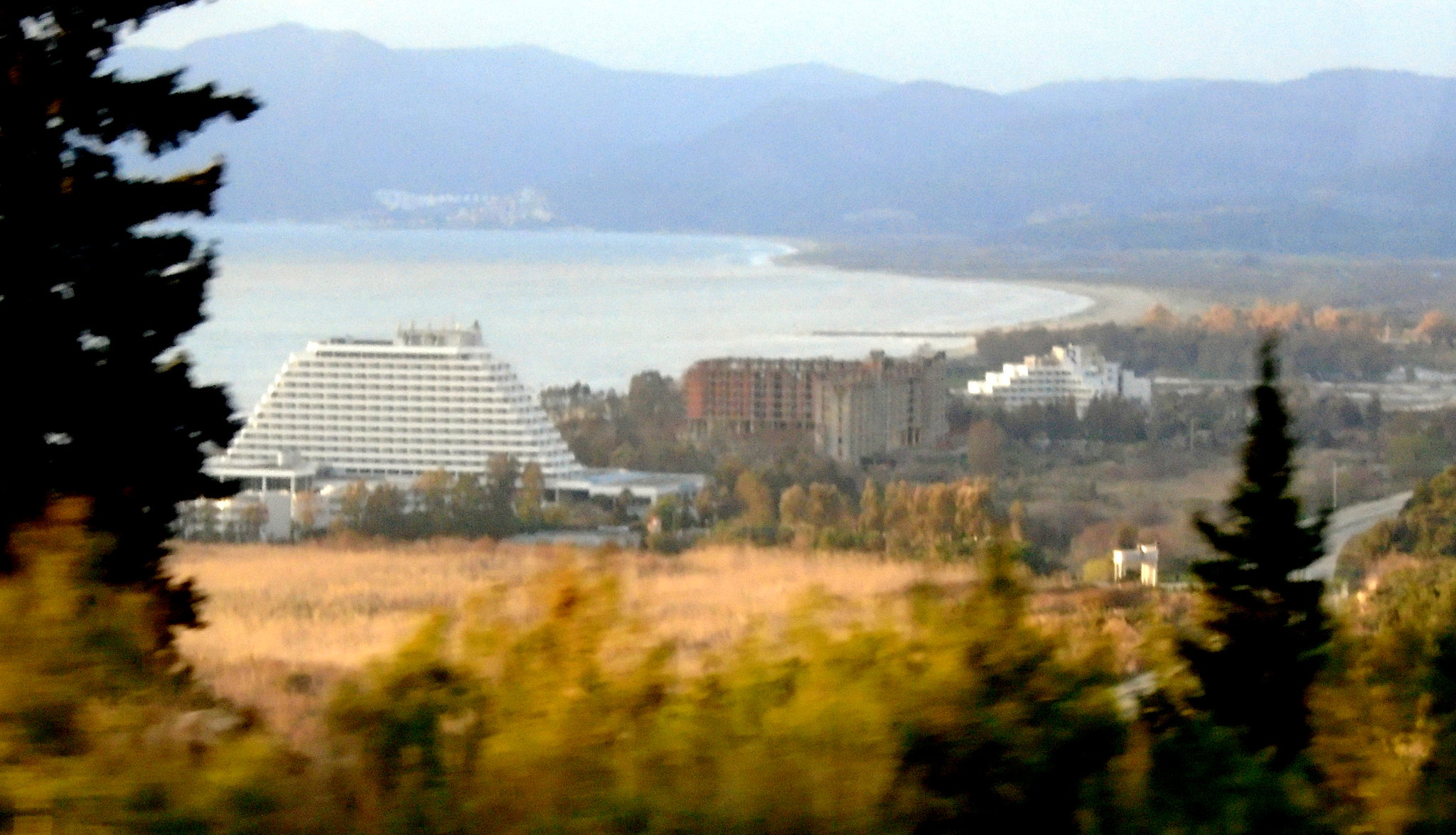This photograph captures a coastal resort city nestled by the ocean with a majestic backdrop of hazy, tree-covered hills. Dominating the scene are three prominent multi-story buildings: a distinctive, trapezoidal white building with numerous windows on the left; a centrally located, brownish-red structure; and another tall, white building further back on the right. The foreground features a mix of evergreen trees and patches of dry, yellow grass, adding texture to the landscape. The ocean stretches into the top left quadrant of the image, its blue hues contrasting against the hazy, blue sky overhead. The image has a foggy quality, lending the city a dreamy, ethereal ambiance, reminiscent of coastal resorts like those in the Bahamas. No people or text are present, focusing all the attention on the natural and architectural beauty of the serene coastal setting.